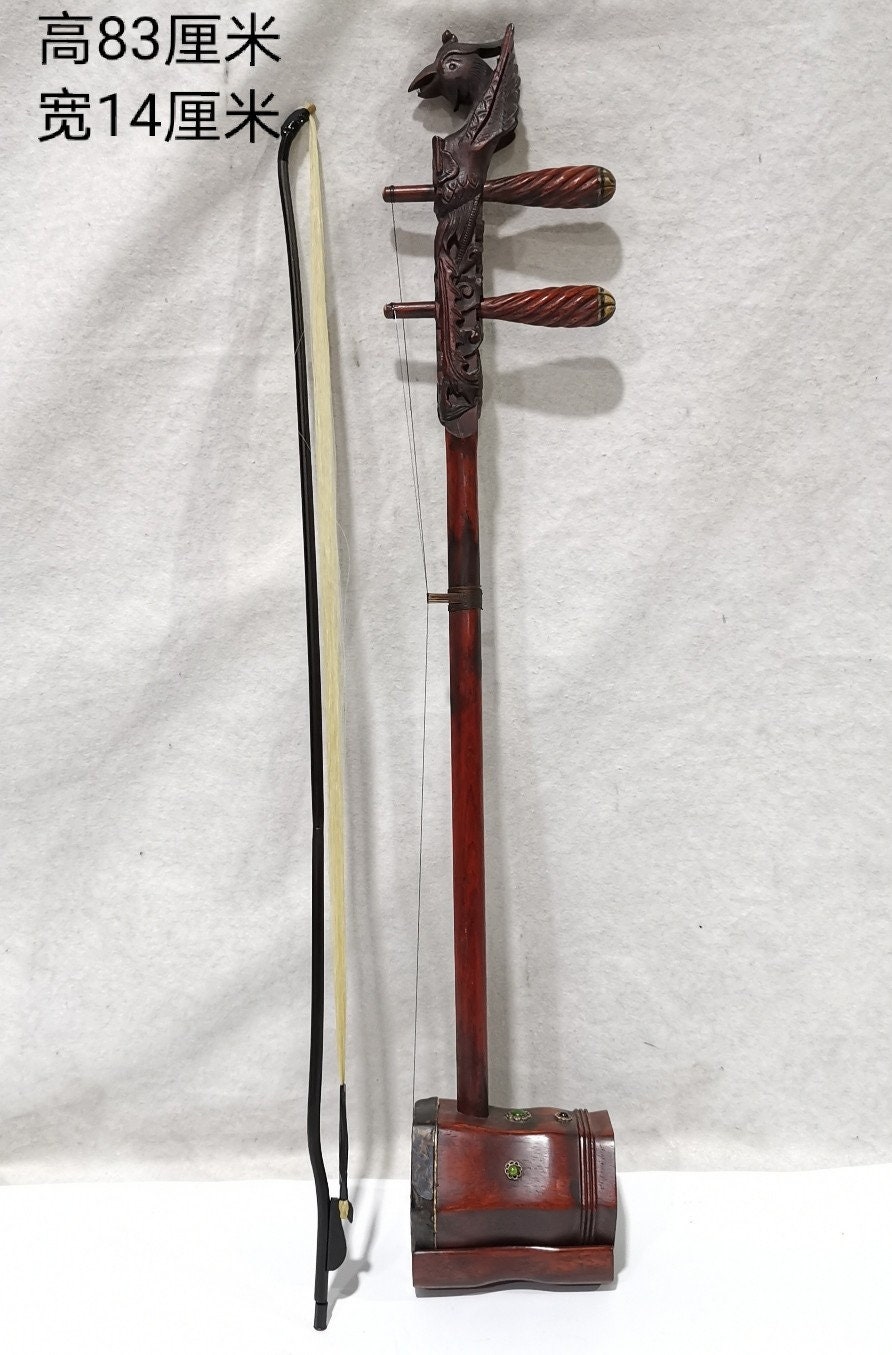The image features an ancient Asian musical instrument, potentially an ancient Chinese proto-violin. The instrument is distinguished by its long wooden neck, which is intricately carved with a bird's head at the top made of darker wood. This bird-like head includes two pegs, used for tuning the single or double strings that stretch to the instrument's bottom, which is shaped like a bongo drum or a small cup. The body of the instrument is adorned with detailed decorations, including gold stars and floral motifs, with green gems at their centers. Accompanying the instrument is a curved bow, possibly made of animal intestine strings. This setup is leaning against a gray or white background, suggesting a display or product shot environment. In the top left corner, there are Chinese characters with the numbers 83 and 14 next to them.